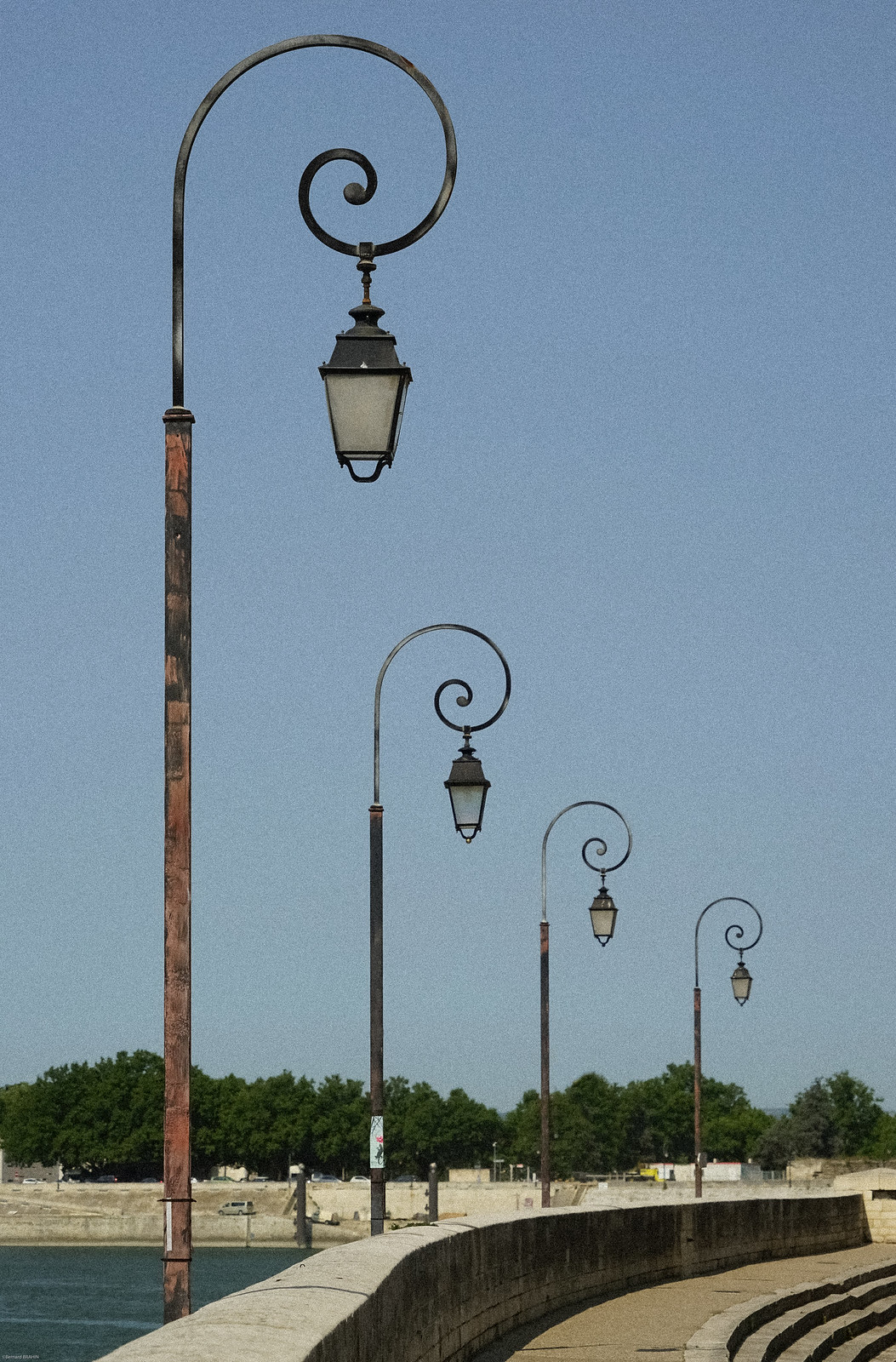The photograph captures a bright daytime scene with a clear blue sky as the backdrop. Clustered in the background are thick trees with dark, deep green foliage. In the foreground, we see a concrete wall with a curve, creating a walkway that overlooks a body of water situated between two parallel concrete barriers. There are four old-fashioned lampposts made of wrought iron, each adorned with a glass-paned lantern hanging from a curved, spiral design at the tops. These lampposts are tall and provide a classic, aesthetic appeal to the scene. Just beyond the lampposts are four concrete steps that ascend to the walkway area where the lampposts stand. Parked cars can be seen near this area, adding a touch of urban life to what appears to be a scenic walking path or bridge adjacent to a river.